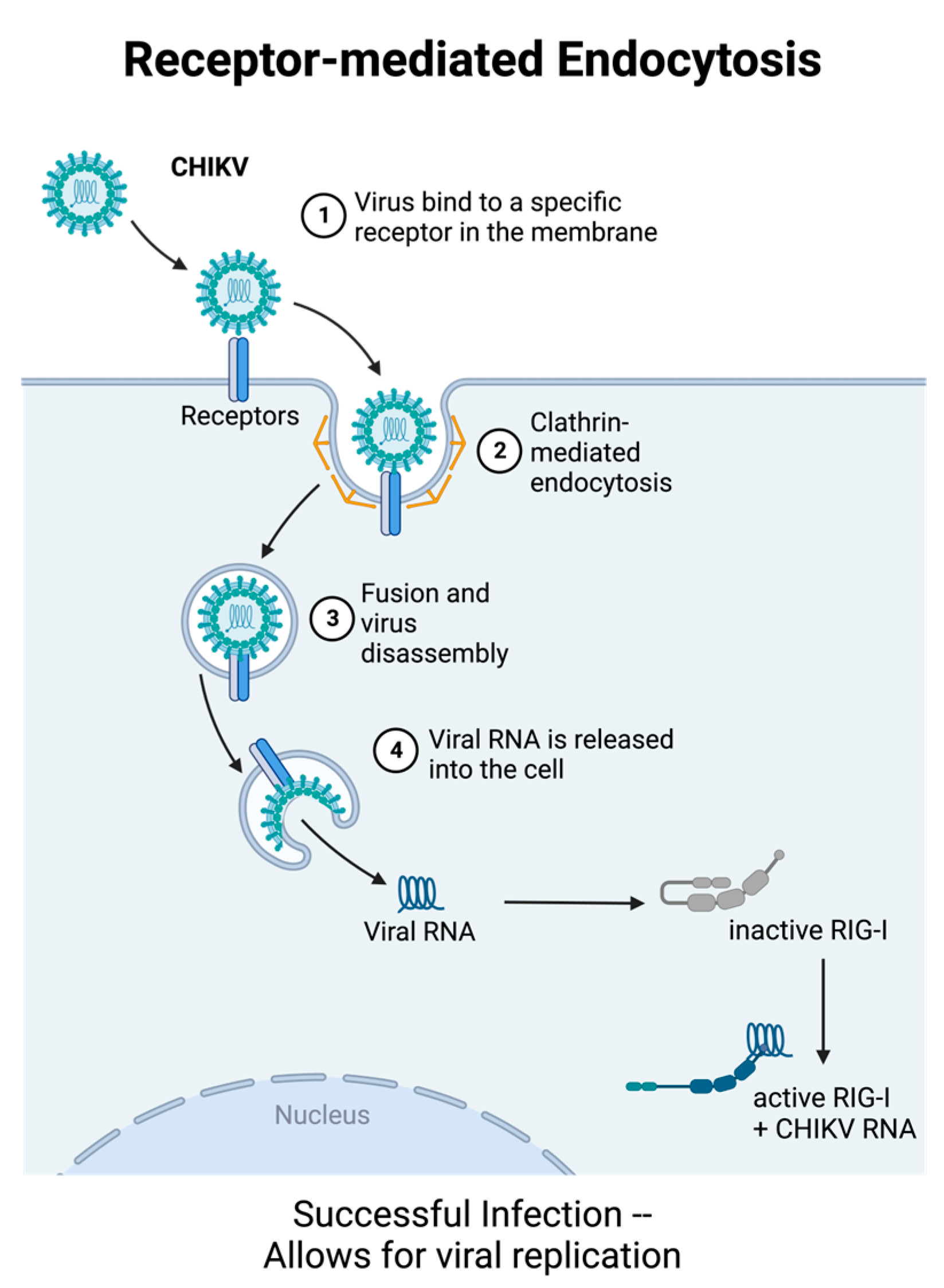This detailed illustration depicts the process of receptor-mediated endocytosis with a focus on viral infection and replication within a medical context. At the top of the diagram, it outlines several sequential steps beginning with a virus, labeled C-H-I-K-V, binding to a specific receptor on the cell membrane (Step 1). The virus is shown as a teal-colored entity with spikes, resembling a coronavirus. Following this, the process of clathrin-mediated endocytosis (Step 2) is highlighted, wherein the cell membrane engulfs the virus, forming an enclosed vesicle. 

Step 3 illustrates the fusion of the virus with the vesicle membrane and the subsequent disassembly of the viral structure. Inside the cell, viral RNA is released (Step 4), depicted as migrating from the vesicle into the cytoplasm. The viral RNA then interacts with inactive RIGI, transforming into active RIGI plus C-H-I-K-V RNA, a step crucial for successful viral replication. The text below the diagram concludes by stating "successful infection allows for viral replication," emphasizing the end result of the depicted process.

Throughout the illustration, the transitions between each step are marked and visual elements like symbols, spirals, and curved pathways visually guide the viewer, providing a comprehensive understanding of how C-H-I-K-V infects a cell and initiates replication.